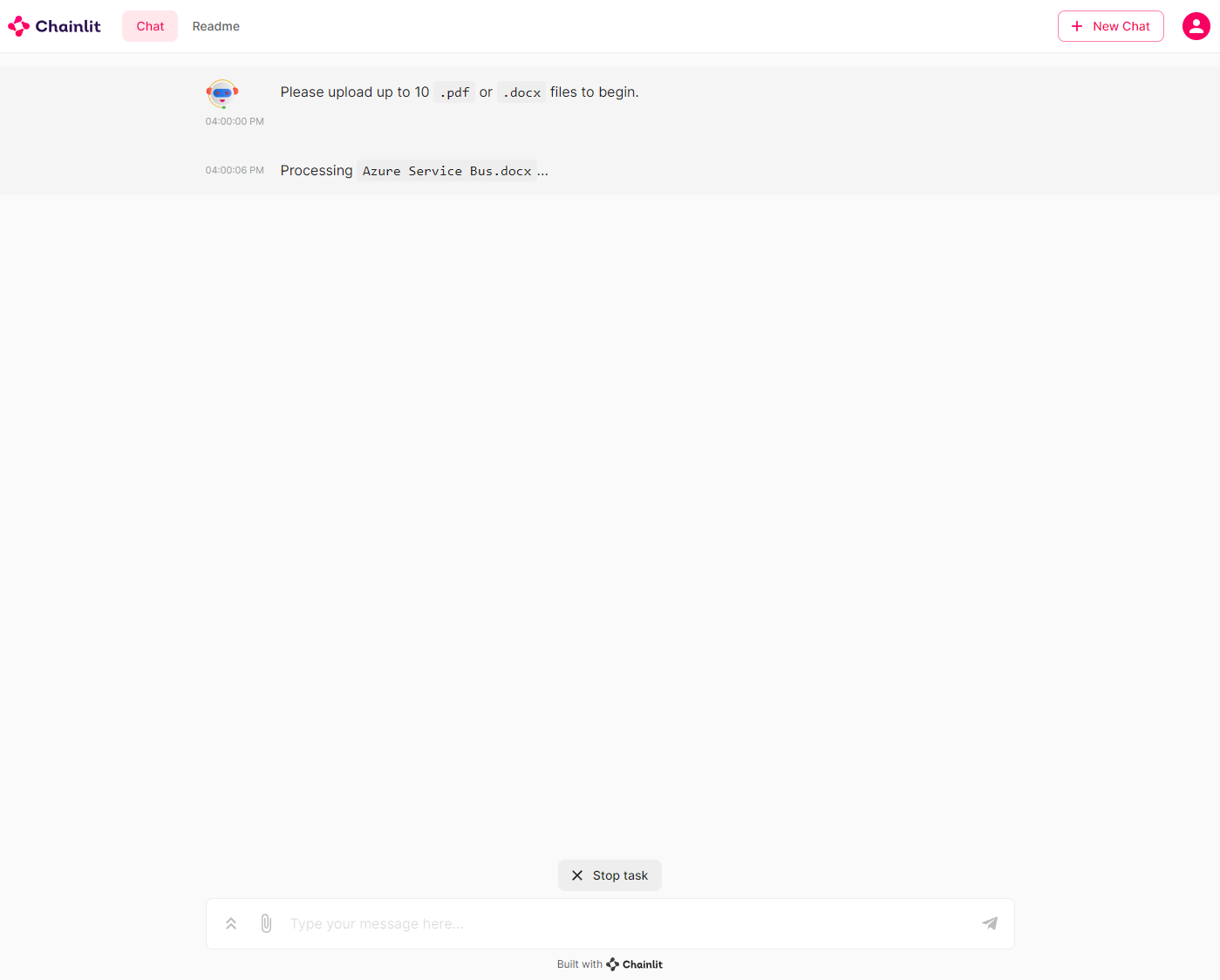The image features a user interface dominated by a purple-themed color scheme. In the top left corner, there is a purple logo resembling a cross with a white center, and the word "ChainLit" written in bold black text. Adjacent to the logo, there is a light purple-colored box with the text "Chat" displayed in dark purple. To its right, "Read Me" is written in black.

On the far right side, a white button with a plus sign labeled "New Chat" is also prominently visible in purple. There is a generic profile picture depicted in a default purple color scheme with a gray box beneath it, instructing users to "Please upload up to 10 PDF or .doc files to begin." This section indicates an ongoing process with Azure services.

Below this, there is a button marked with an "X" and the text "Stop Task." Lastly, at the bottom of the interface, there is a text box with a prompt stating "Type your message here," and the phrase "Made with ChainLit" is clearly displayed.